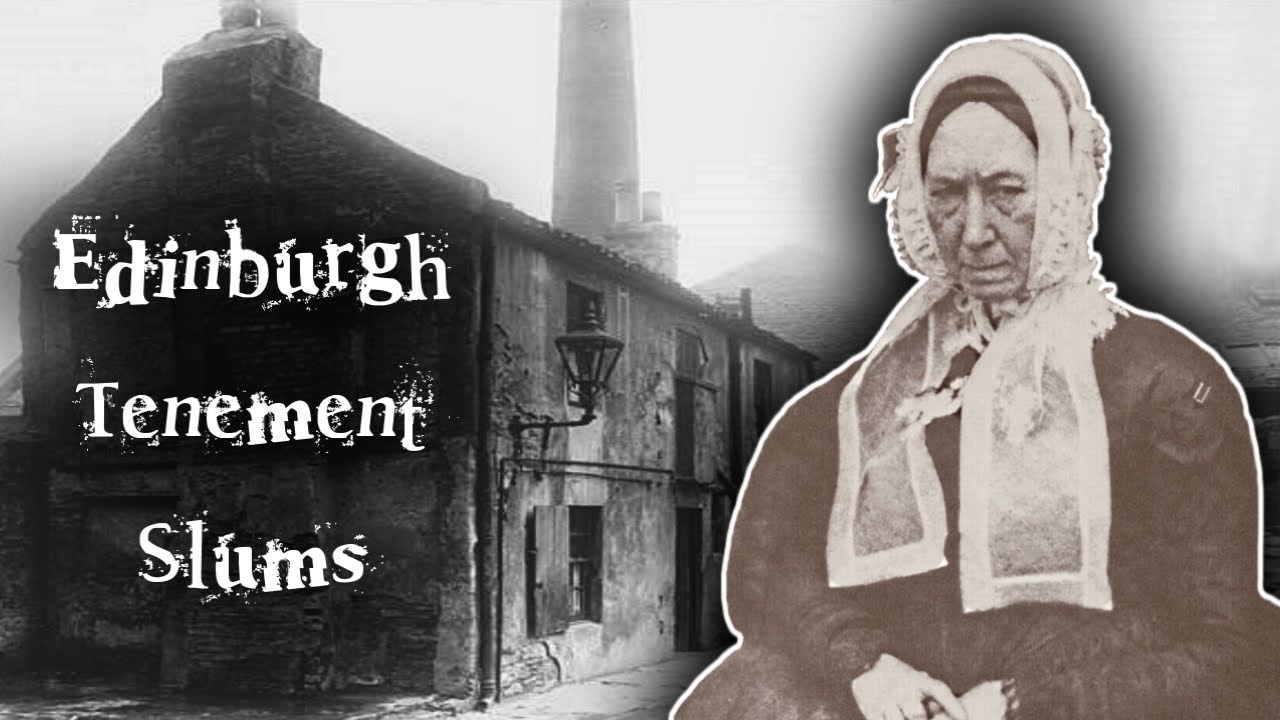This intricate composite image merges two vintage photographs to create a compelling visual narrative. The background is a black-and-white photograph depicting old, dilapidated tenement buildings in Edinburgh. These two-story structures, adorned with lanterns, exude an aura of neglect, their exteriors weatherworn and deteriorated. Various chimneys punctuate the rooflines, including a particularly tall one standing prominently in the distance. The sky overhead is a murky grey, suggesting a foggy atmosphere that enhances the setting’s bleakness. Along the edge of the leftmost building, the words "Edinburgh Tenement Slums" are emblazoned in an eerie, horror-movie-inspired font, complete with splatter motifs, adding a layer of grim melancholia.

Superimposed on the right-hand side of this scene is a stern-faced older woman, digitally cut out from another photograph. She is adorned in a somber black dress with a high collar, a stark contrast to her white bonnet. The bonnet is detailed with two long white pieces that drape over her shoulders and chest, further emphasizing her austere appearance. This juxtaposition of imagery creates a haunting tableau that speaks to the hardships and historical context of life in the Edinburgh tenement slums.